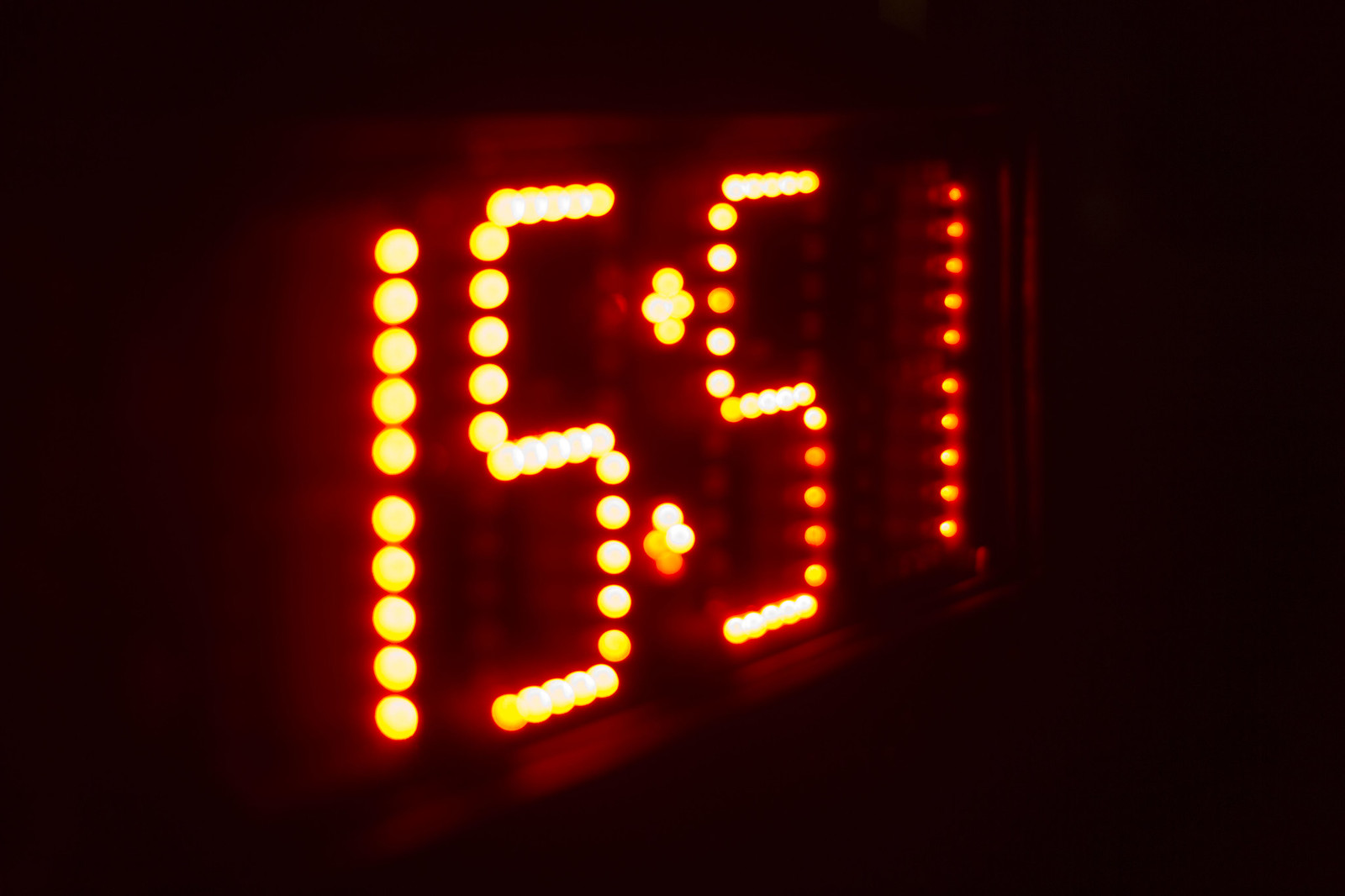This photograph, taken in low-light conditions or possibly at night, features a digital clock displaying the time "15:51". The clock is a large, rectangular device, oriented with its left side pointing towards the bottom left corner of the image and its right side positioned more centrally. The illuminated digits emit a captivating blend of white, yellow, and orange hues. The '1' in "15" is depicted with a unique formation of 10 dots: 5 dots at the top, a small gap, and 5 dots at the bottom. Meanwhile, the '5' and '1' of "51" are similarly constructed from a grid of glowing dots. The colon separating the hours from the minutes consists of a vertical arrangement of four dots, further enhancing the clock's digital aesthetic.